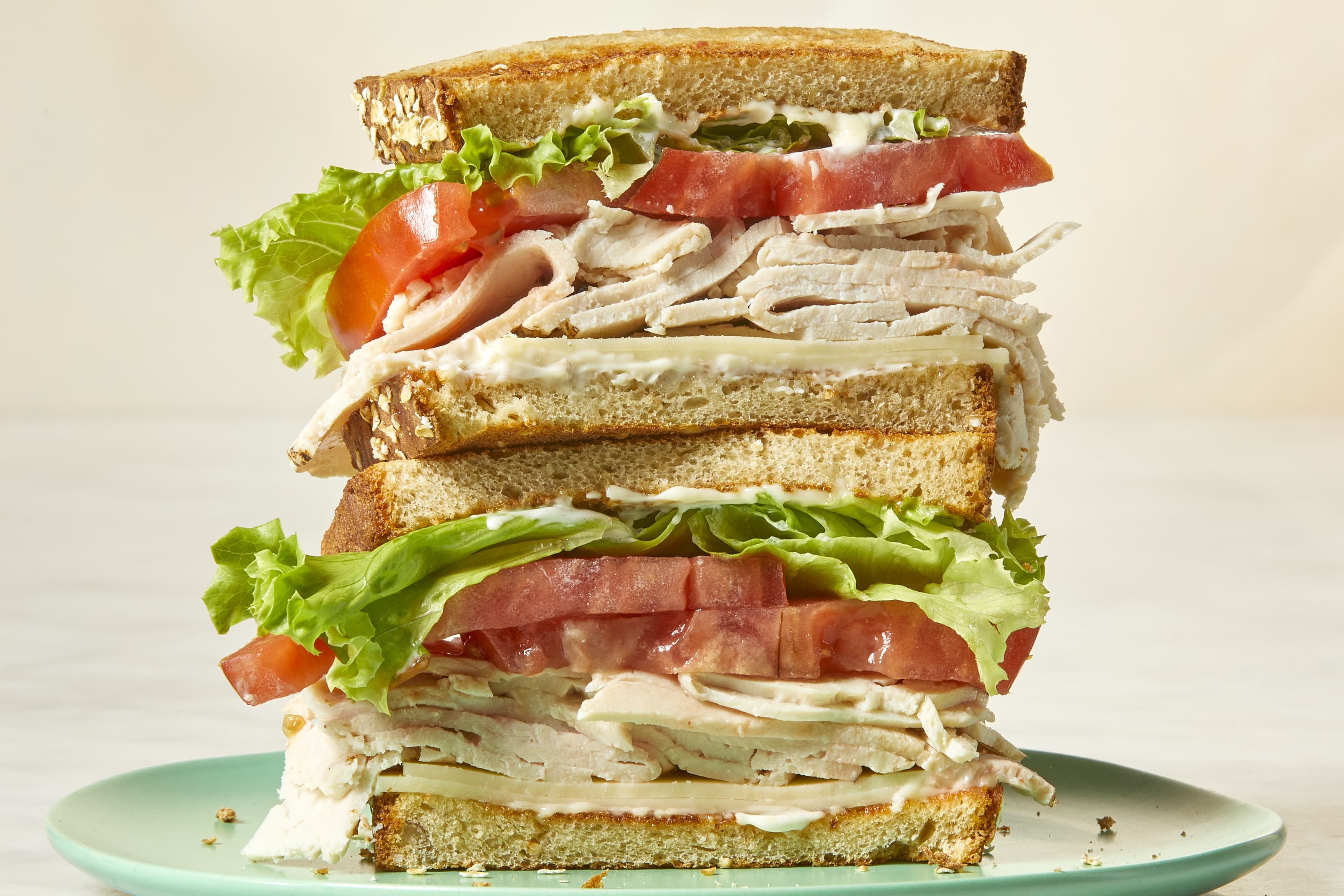This detailed photograph captures a mouth-watering turkey, tomato, and lettuce sandwich with layers of ingredients that create an appetizing visual. The sandwich, stacked to resemble a club sandwich, features two halves perched one on top of the other. Each half showcases thickly cut, juicy red tomato slices, a generous amount of folded turkey, crispy lettuce, and slices of pale white cheese, all richly coated with thick mayonnaise. The ingredients are layered neatly between what appears to be toasted wheat bread, exhibiting a slight brown, burnt texture. The sandwich is presented on a light green ceramic plate, speckled with a few bread crumbs, and set against a white table or marble surface. The background of the image subtly shifts to a pinkish hue, hinting at a distant wall. The entire presentation emphasizes the sandwich's substantial size and the abundance of its fresh ingredients.